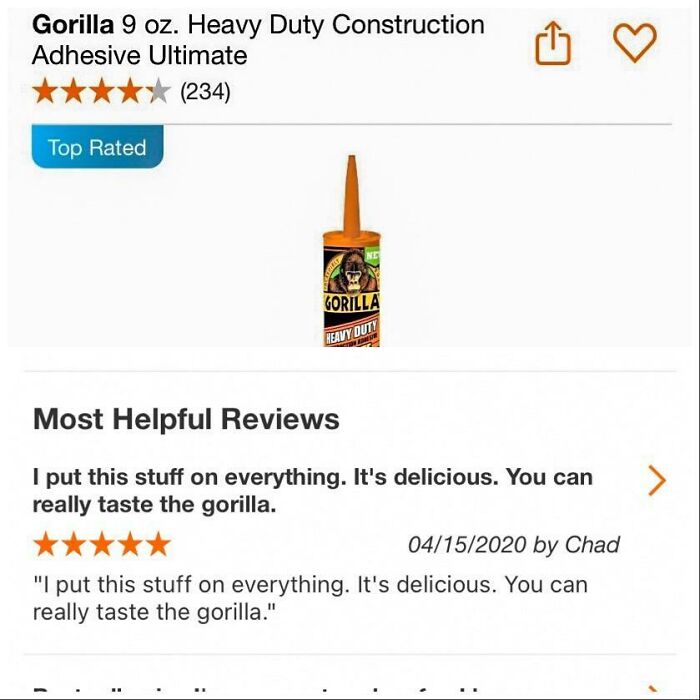The image showcases a product advertised as "Gorilla 9oz Heavy-Duty Construction Adhesive Ultimate." The packaging prominently features the iconic Gorilla logo, with the word "Gorilla" displayed boldly. The adhesive comes in a tube with an orange tip. The product has received an overall rating of 4.5 stars based on 234 reviews. There are various interface elements depicted, including an orange square with an up arrow icon, an orange heart, and a blue square.

Below the product image, there is a highlighted review titled "Most Helpful Reviews." The review, dated April 15, 2020, is given by a user named Chad. Chad rates the product 5 stars and humorously comments, "I put this stuff on everything, it's delicious, you can really taste the Gorilla." The review text is repeated for emphasis. Surrounding the text are borders and lines that add to the visual structure of the advertisement.

Overall, the image is carefully designed to emphasize the strong branding and positive customer feedback, likely aiming to attract and reassure potential buyers.